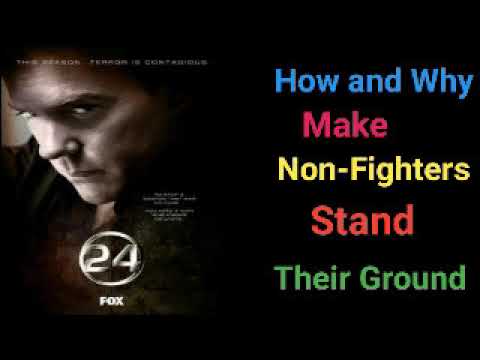The image is an advertisement for the TV show "24," prominently featuring a poster of Jack Bauer, the show's lead character, on the left-hand side. The poster presents a close-up of Jack Bauer's contemplative face, with him glancing downward. The title "24" is displayed in silver within a circular silver ring, and the word "Fox" is positioned below the logo, denoting the network airing the show. The background of the poster is solid black. Adjacent to this on the right-hand side, there is colorful text that reads, "How and why make non-fighters stand their ground." The arrangement groups the words by color: "How and why" in blue, "make" in red, "non-fighters" in yellow, "stand" in orange, and "their ground" in green. Despite the prominence of these phrases, there seems to be no clear connection between the content of "24" and the message about making non-fighters stand their ground. The only legible text on the poster declares, "This season, terror is contagious."